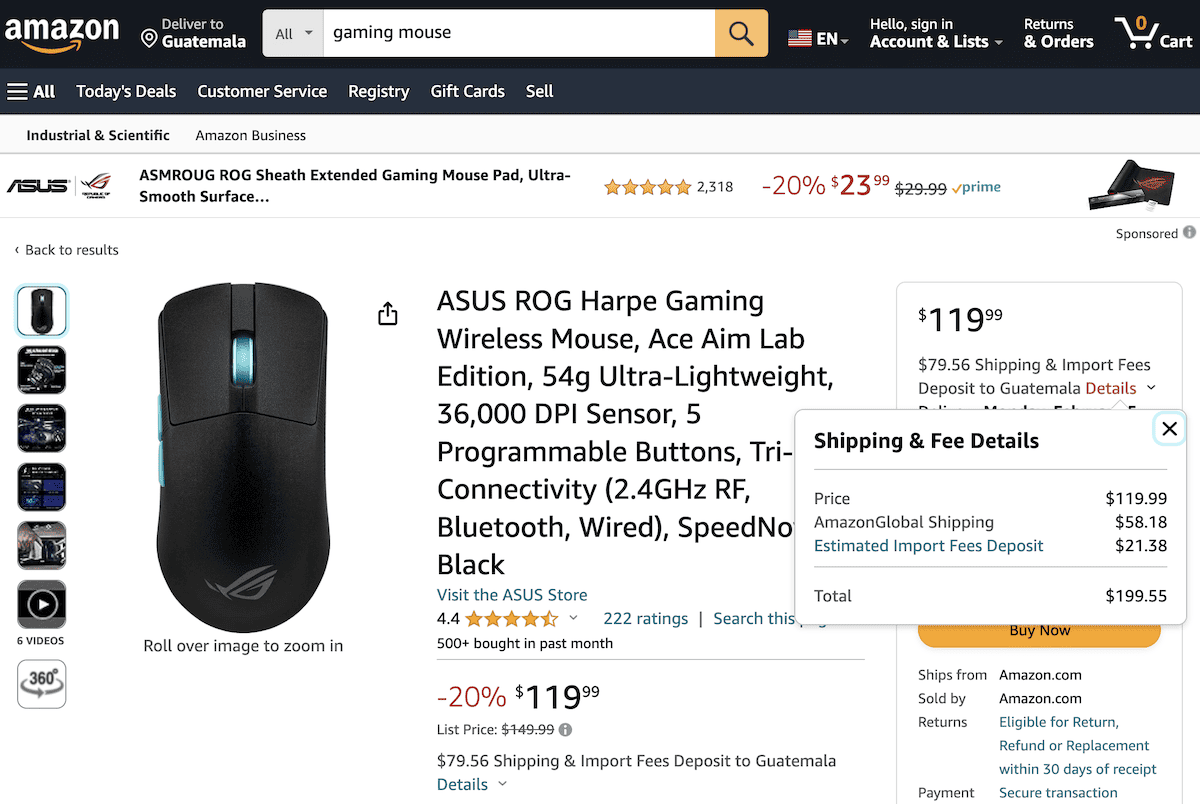This detailed screenshot from Amazon showcases a search result for an Asus ROG Harp Gaming Wireless Mouse. The familiar Amazon logo is positioned on the left, and the interface is in English. The screenshot indicates that the item has been delivered to Guatemala. The Amazon navigation bar includes options such as "Hello, sign in," "Accounts & Lists," and "Returns & Orders."

The product in focus is the Asus ROG Harp Gaming Wireless Mouse - Ace Aim Lab Edition. This high-performance mouse is distinguished by its ultra-lightweight design of just 54 grams, featuring a 36,000 DPI sensor, five programmable buttons, and tri-connectivity options (2.4GHz RF, Bluetooth, and wired). It is available in black and directs users to "Visit the Asus Store" for additional products and information.

The customer ratings show a strong approval, with the mouse earning 4.4 stars from 222 ratings, and it is noted that 500 units were purchased in the past month. The product is offered at a 20% discount, reducing the price to $119. However, international shipping and import fees for delivery to Guatemala amount to $79.56, bringing the grand total to $199.55.